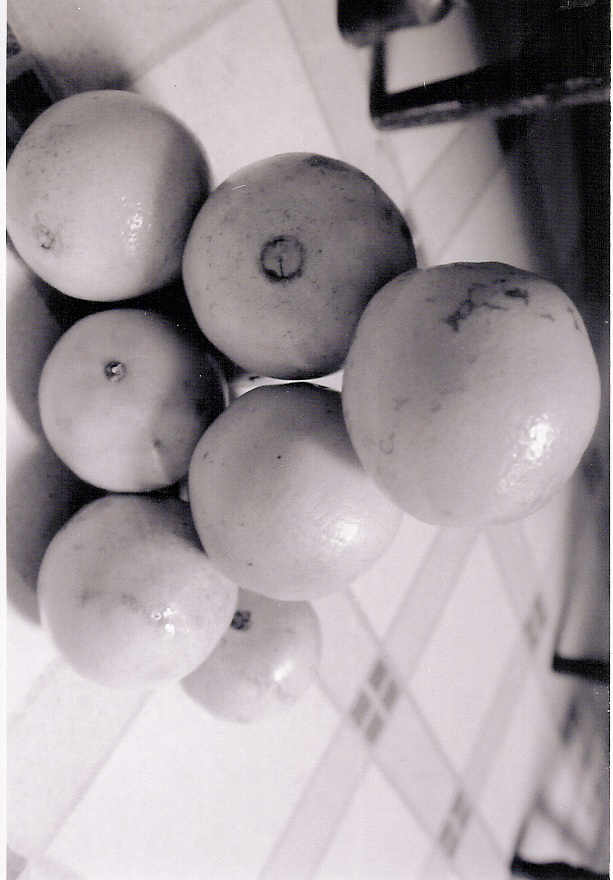This black and white image, rotated 90 degrees to the right, depicts a stack of oranges arranged into a pyramid on a linoleum floor with an old-fashioned checkered pattern. The grid consists of larger squares, each framed with intersecting lines, and smaller squares at the center of each four-square intersection. The pyramid of oranges is composed of three at the bottom, two in the middle, and one at the top, with an additional orange lying behind and slightly to the right, partially peeking out two-thirds from behind the stack. The fruits, likely oranges due to their size, appear pale in the grayscale photo. In the background, towards the left and right edges of the image, there are dark wooden chair legs touching the floor, reinforcing the notion that the oranges are indeed on the floor. The lighting highlights portions of the oranges, adding depth to the scene.